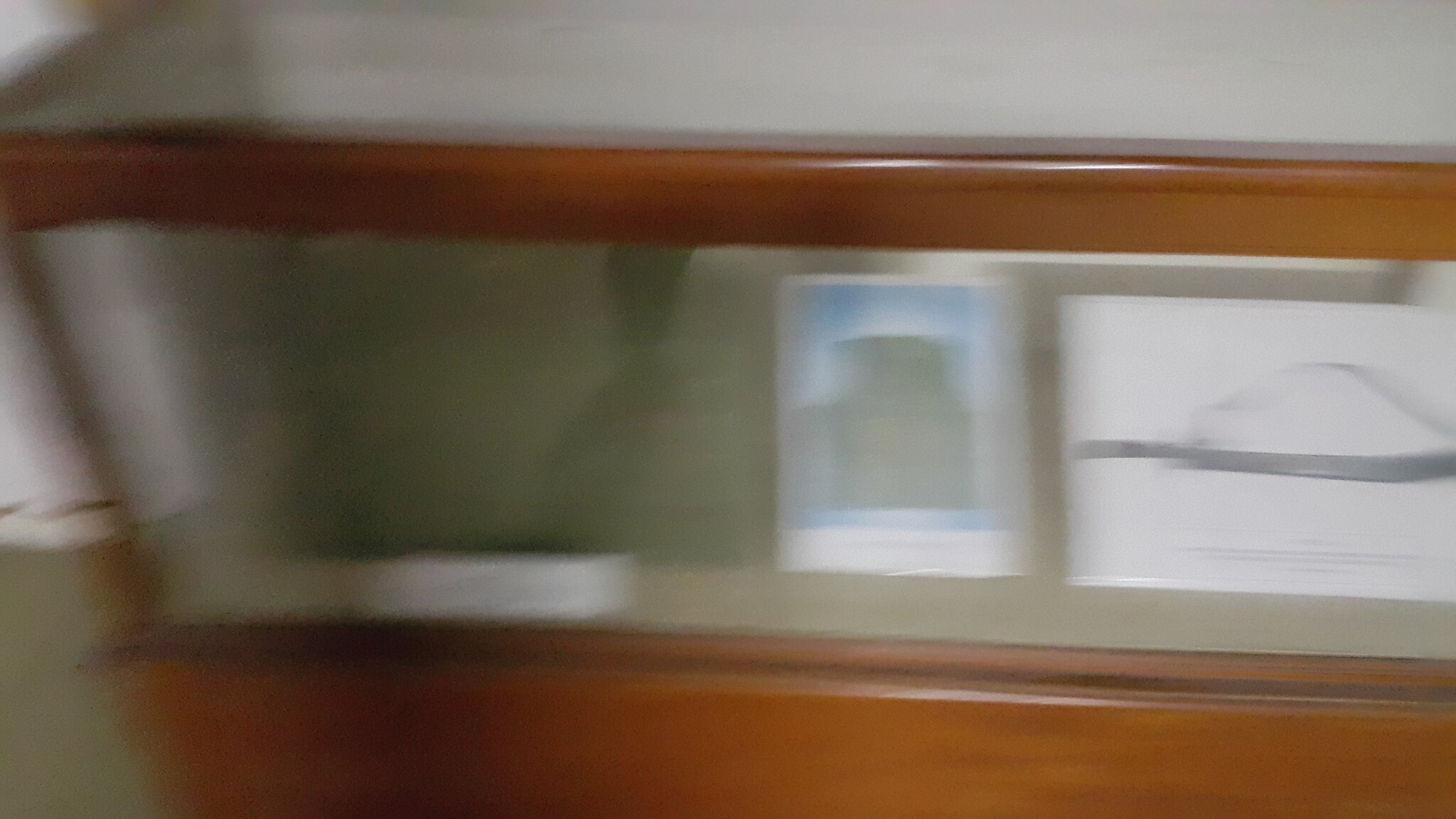The image is noticeably blurry, making the details difficult to discern. However, it seems to depict a museum display or a decorative shelf possibly situated in an exhibit. The central object appears to be a wooden piece of furniture with a sophisticated design suggestive of a vintage or handcrafted item. The structure is primarily rectangular and bordered with a warm, orangey-reddish wooden frame. The top and all four sides are enclosed with glass, providing a transparent view of the interior, which is supported by a sturdy wooden base.

Inside the display case, there appear to be three distinct objects. The first resembles an image or a sculpture depicting incense burning, exuding an aura of tranquility. The second object seems to be a square-shaped item, possibly another picture or artifact. Additionally, there are two unclear objects that look like plant images or actual plants, adding a touch of nature to the display. The left side of the image is particularly blurry, making it challenging to identify specific features, but a white base is noticeable amid the haze.

Despite the blurriness, the display's elegant design and the intriguing mix of objects hint at a carefully curated collection intended to draw the viewer's interest and curiosity.